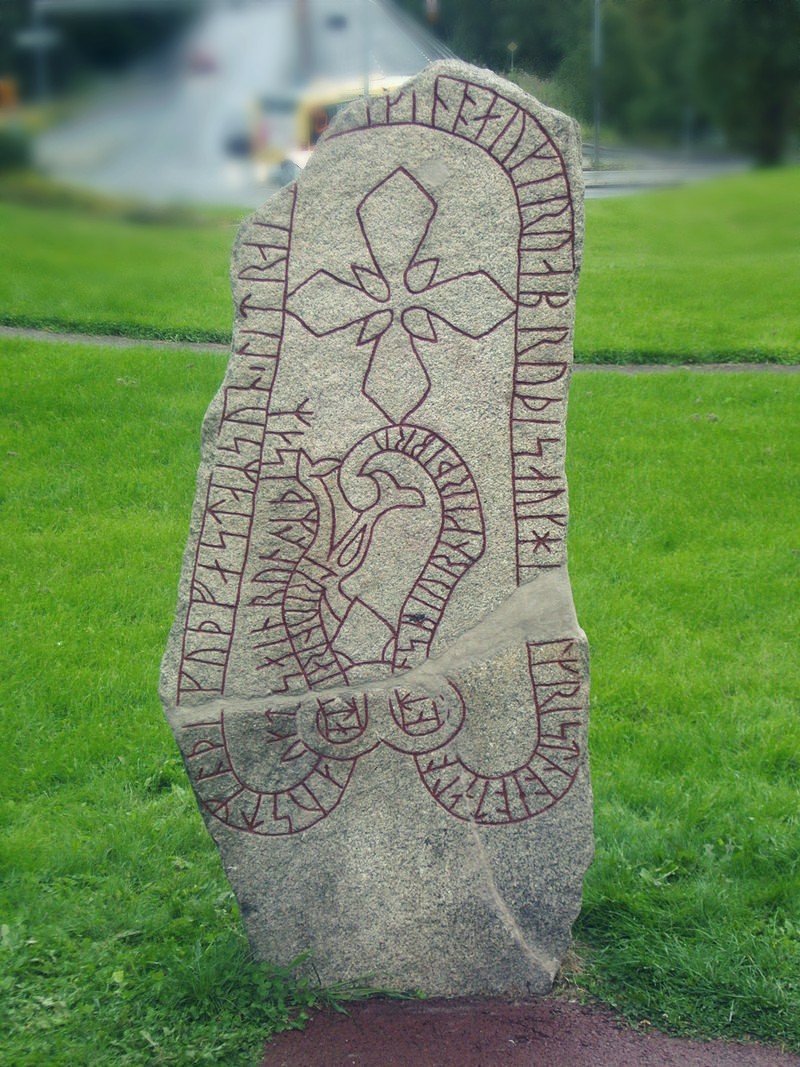In this outdoor photograph, a tall grey stone pillar stands prominently amidst a lush, dark green grassy field. The pillar, flat on its front surface, is adorned with intricate red-hued carvings that depict elaborate designs. Along the edges of the stone are serpentine shapes, reminiscent of snakes winding towards the center. These snake-like carvings enclose several symbols, which may represent letters or other significant marks. At the top center of the stone, a diamond-shaped cross is visible, while towards the lower section, a figure-eight shape can be seen, resembling an eye mask connecting different segments. The stone monument, standing on a slightly reddish stone base, is part of a hazy background where details blur into the distance.